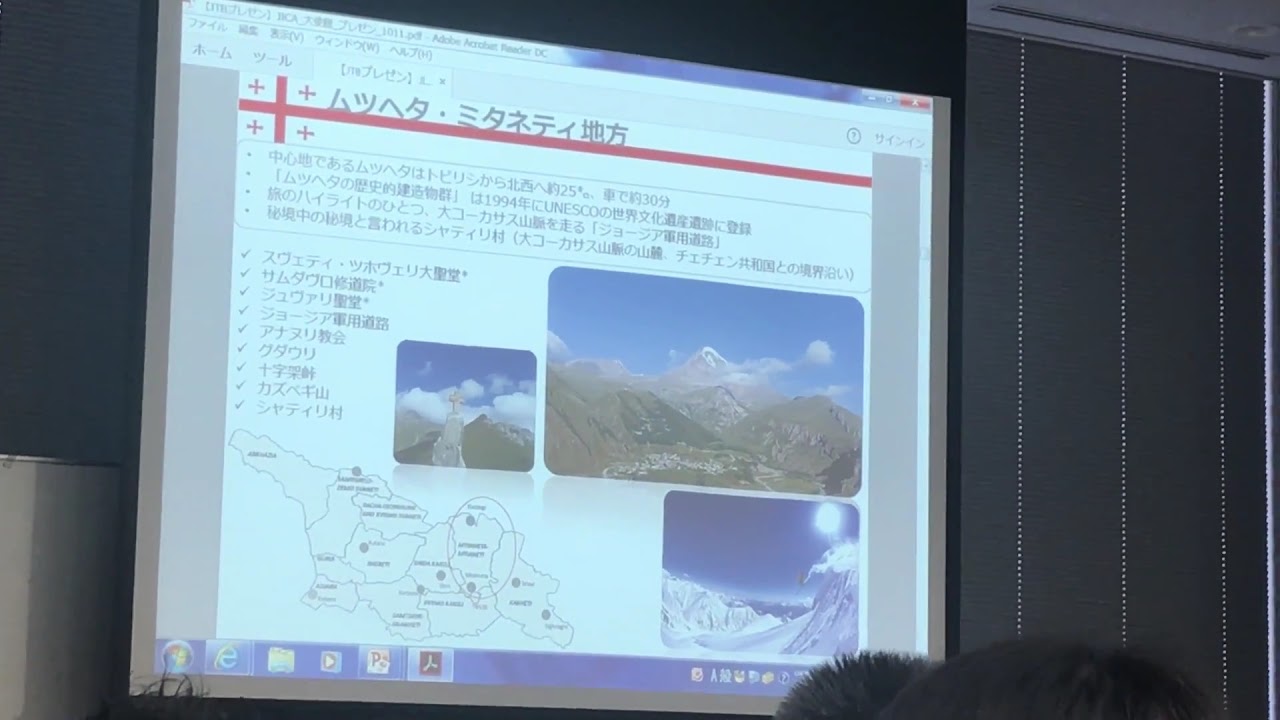The image shows a projected PowerPoint slide or a large monitor display, featuring detailed content written in what appears to be Asian characters, likely Japanese. The slide is set against a grayish background with dotted lines and white trim along the ceiling, suggesting it's displayed in a dimly-lit room with closed windows on the right. The slide includes a variety of visuals: on the far left, there is a map that could symbolize directions or a travel route. To the right of the map, there are images of mountains—some snowy and others lush with greenery. Below, there's a cliff or similar geological feature. Additional icons at the bottom left of the screen include Adobe, Internet Explorer, Windows, File Explorer, and Windows Media Player, indicating that this might be a computer screen image or screenshot. The lower right corner of the image partially shows what seems to be a fuzzy object, possibly someone's head or hat. Overall, the setup and the presence of presentation software and icons suggest this is an informative or travel-oriented slide being shown in a modern setting.